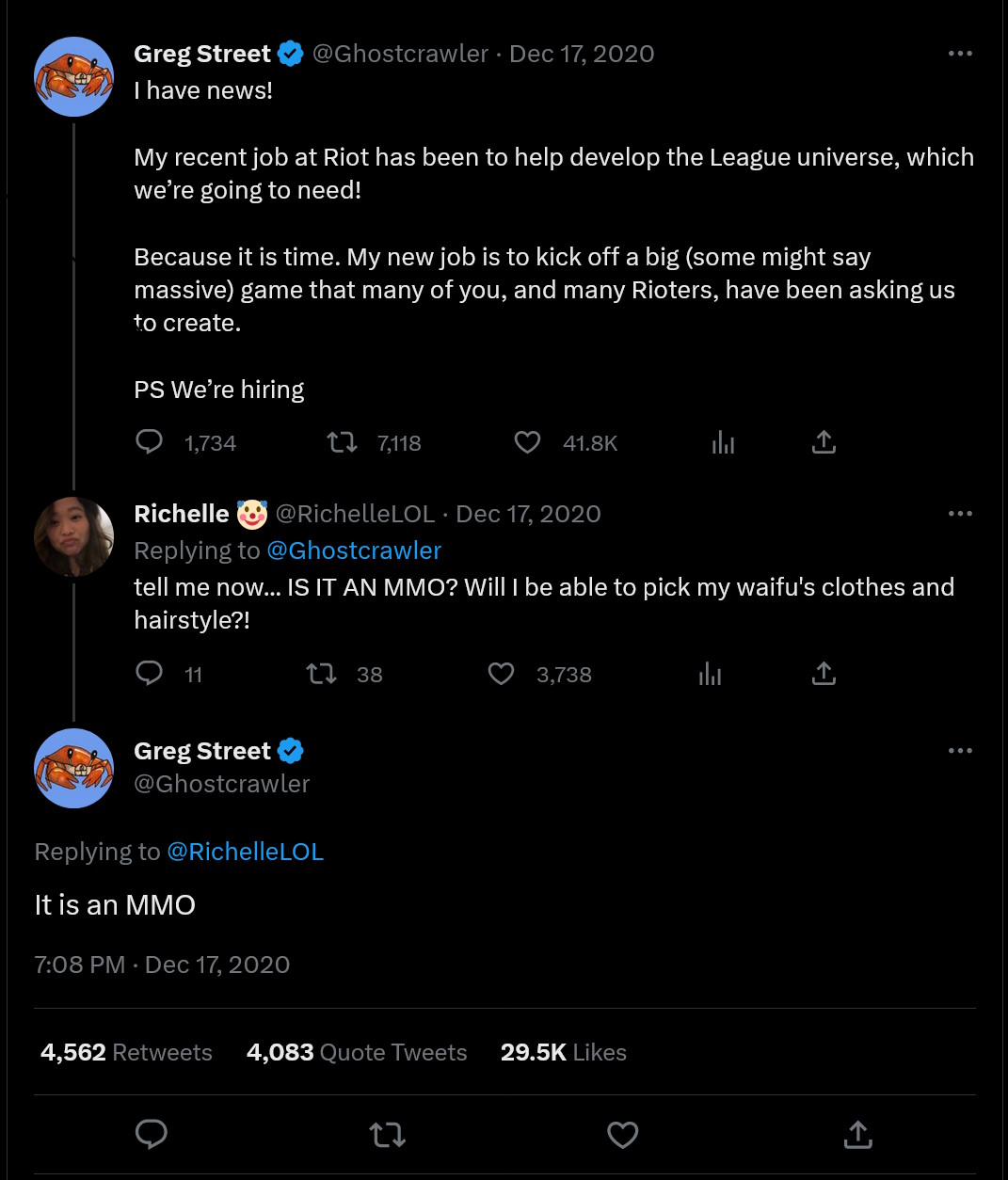Screenshot of a Social Media Conversation about a New Game Announcement

Description: This screenshot captures a riveting exchange on social media. The background is black, with the majority of the text appearing in white, interspersed with some blue highlights. At the top, the conversation begins with a post from Greg Street, indicated by a blue circle icon featuring a red crab. Greg's profile is verified, denoted by the blue checkmark next to his handle, @Ghostcrawler. His post, dated December 17, 2020, starts with an enthusiastic "I have news!" 

In his message, Greg announces his recent role at Riot Games, working on the League universe, and reveals an exciting new project: a massive game that Riot and its community have been eagerly anticipating. He caps off his announcement with a call for recruits, stating "P.S. We're hiring." The post has garnered significant engagement, evidenced by 1,734 comments, 7,118 shares, and an impressive 41,000.6 likes.

Below Greg's post, a user named Rachelle responds. Her profile picture shows an Asian woman with brown hair, and her handle is @RachelleLOL. Responding to Greg’s announcement, she eagerly inquires, "Tell me now, is it an MMO? Will I be able to pick my waifu's clothes and hairstyle?" Her post, also dated December 17, 2020, has attracted 11 comments, 38 shares, and 3,738 likes.

Greg replies to Rachelle’s question, confirming, "It is an MMO." This reply, timestamped at 7:08 PM on December 17, 2020, further stirs excitement among the followers, resulting in 4,562 retweets, 4,083 quote tweets, and 29.5k likes.

At the bottom of the screenshot, four icons are visible: a conversation bubble for comments, a retweet icon, a heart for likes, and an arrow with a bracket, presumably for sharing the post elsewhere.